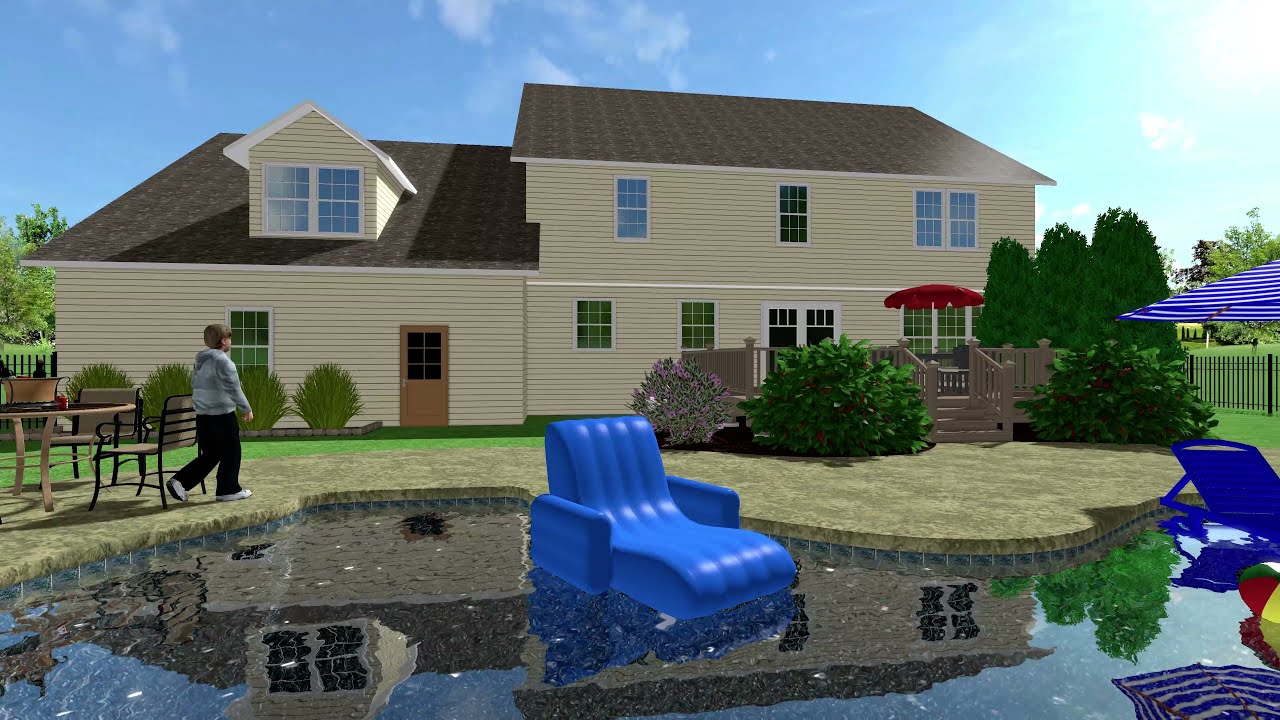In the backyard of a large, two-story house with beige or light-yellow siding and a brown roof, a diverse scene unfolds beneath a partly cloudy blue sky. The house, featuring numerous windows, has a small deck with steps on its right side and a visible doorway on the left. 

In the foreground, a shimmering pool takes center stage, adorned with two blue floating chairs and partially obscured blue-and-white striped umbrella reflections dancing on the water. Nearby, a possible ball adds a playful touch to the scene. 

On the left side of the image, a young boy dressed in a gray coat and black pants walks towards the house. Beside him, there’s an outdoor table flanked by two brown chairs, offering a cozy spot for relaxation. A grassy area and several deciduous trees dot the surroundings, adding to the backyard's inviting and tranquil atmosphere.